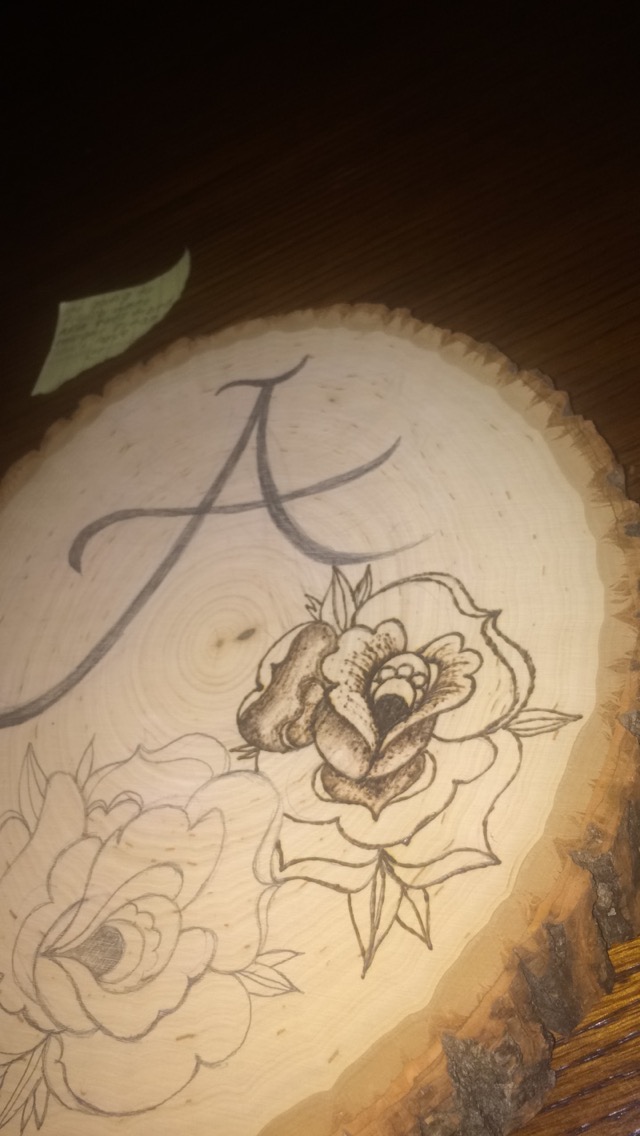This detailed image showcases a partially drawn artwork on a cross-cut oak stump, revealing intricate textures of both the tree's grain and bark. At the top center of the circular stump, there is a meticulously crafted capital A, adorned with elegant flourishes. Below the letter, two flowers are depicted: the one on the left is a stenciled outline lacking any shading or coloring, presenting a clear and simple beauty, while the flower on the right is partially shaded, displaying a speckled dot technique that adds depth and detail to its dark-centered petals. The stump, with its rich hues of brown bark that transitions to a lighter wood inside, anchors the artwork, creating a natural canvas that blends art and nature seamlessly. Additional elements such as tree texture and burn marks enrich the visual experience, and a sticky note rests at the upper left corner of the image, adding a touch of casual realism to the meticulously detailed scene.